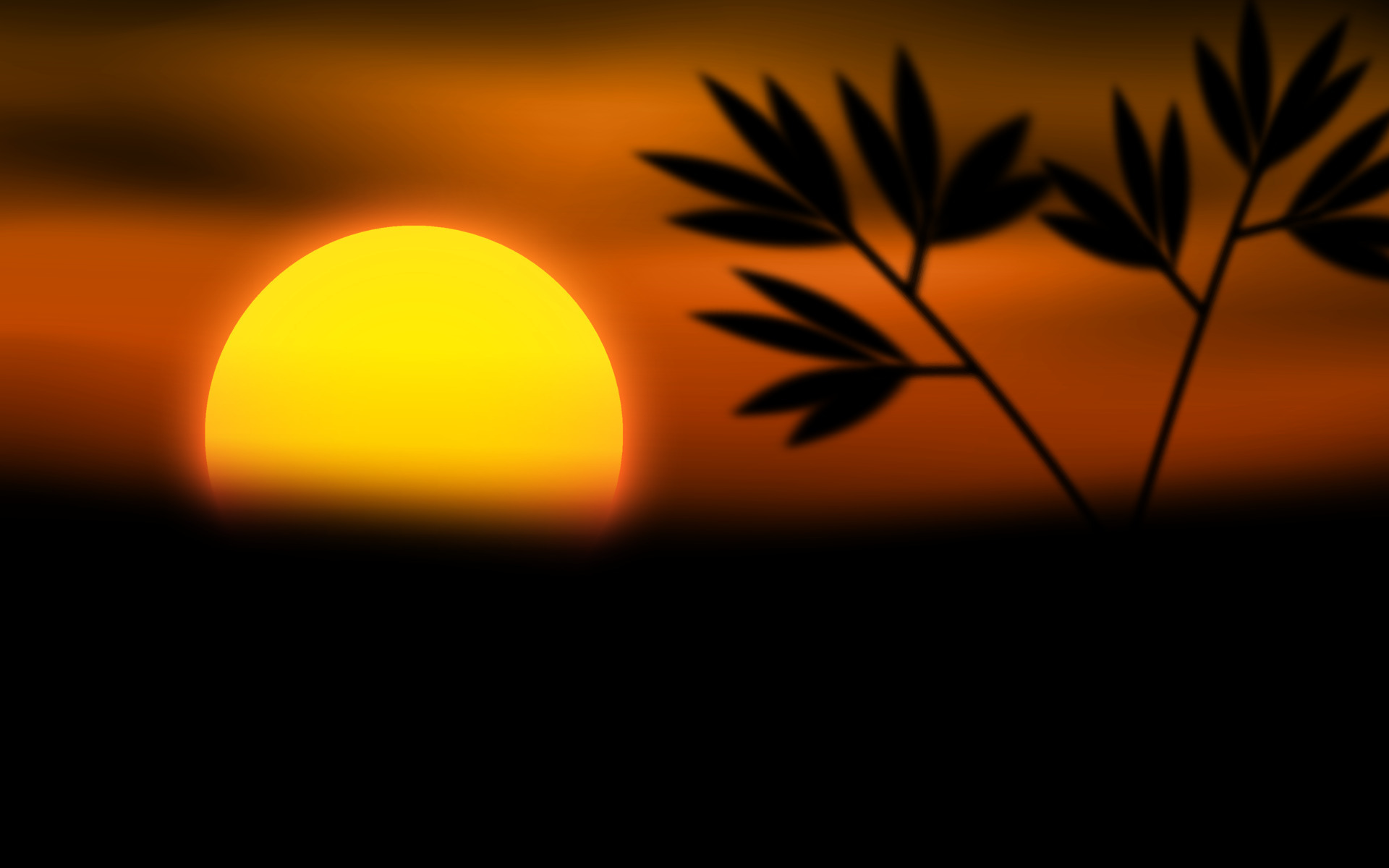This outdoor image captures a serene sunrise or sunset, where the sky is painted in rich shades of orange with streaks of black clouds. The sun, slightly left of center and midway from top to bottom, is a smooth, bright yellow circle trimmed with orange, peeking over a blurry, solid black horizon that covers the bottom portion of the image. To the right side of the frame, the silhouette of a young plant with two twigs each adorned with three clusters of leaves adds a delicate touch to the scene. The overall composition is soft and unfocused, giving it a gentle, dreamlike quality.